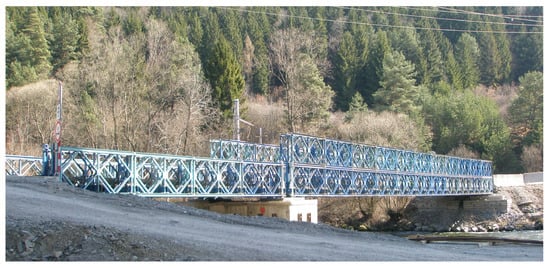The photograph captures an angled view of an intriguing bridge spanning what looks like a rocky, dirt-leveled hill. The bridge, primarily constructed from green-painted steel, features distinctive metal boxes with triangular patterns. These boxes are stacked in a double-decker formation, extending from a concrete support pillar at the near end. The bridge’s hue shifts between bluish-gray to a light green color, depending on the section. 

In the foreground, the terrain appears unpaved and consists of gray dirt, creating a stark contrast with the structured metal bridge. The bridge structure is accompanied by concrete barriers and supports, firmly anchoring it. Beneath the bridge, the view opens up to a possible water passage and a hint of a white building amid the detailed infrastructure on either side.

The background presents a forested area comprising a mix of evergreen trees and deciduous trees, the latter either leafless or brown, hinting at seasonal transition. Power lines are visible running through the right side of the image, cutting through the tranquil scene captured in mellow, washed-out colors. In essence, the photograph offers a layered composition of industrial design harmoniously nestled against a rustic, natural backdrop.